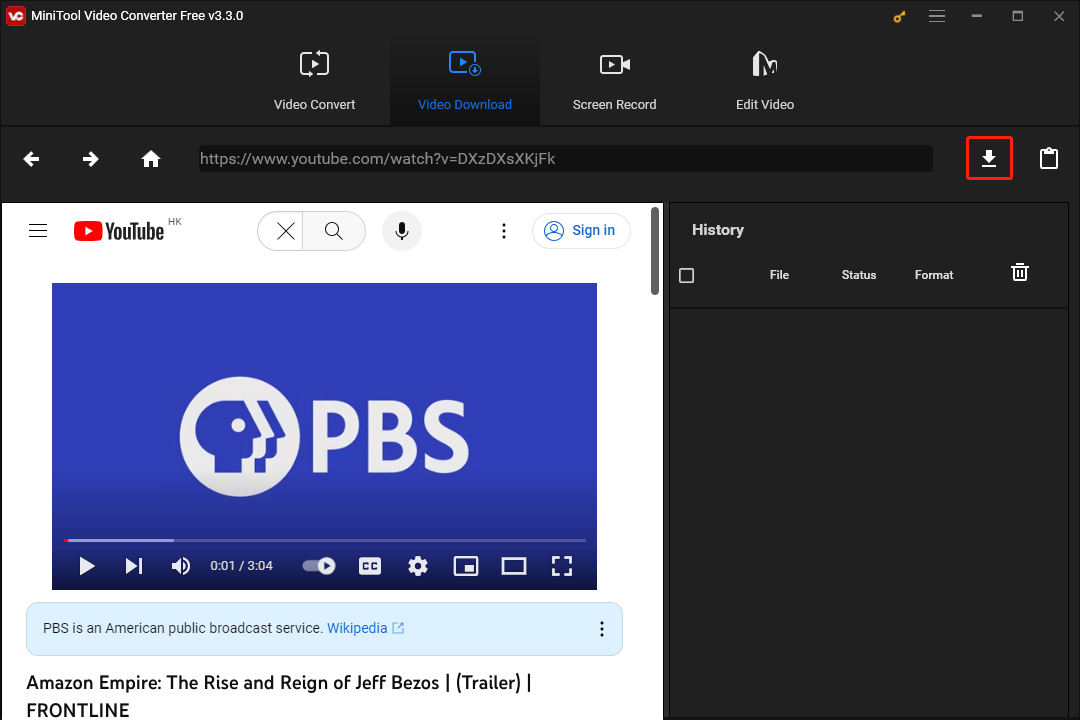The image features a user interface for the "MiniTube Video Converter Free v3.3.0" software. At the top of the application window, the software title is prominently displayed. On the right side, there is a menu bar featuring icons for key functions: menu, minimize, fullscreen, and close (X). Below this are clickable buttons for various actions including "Video Convert," "Video Download" (highlighted in blue, indicating it's currently selected), "Screen Record," and "Edit Video," all displayed in white text.

Directly beneath these buttons is a search or address bar. To the left of this bar are backward and forward navigation arrows adjacent to a home icon, all in white. The address bar is populated with "https://www.youtube.com/watch?v=dxzdxsxkjfk." To the right of the address bar is a download arrow icon surrounded by a red square, and next to it, a clipboard icon.

Below this section, there's a black area labeled "History" in white letters, containing a white square. This area includes various fields named "File," "Status," "Format," and a trash can icon. To the left of this section, there is a small display area showing a YouTube interface. This segment includes the YouTube logo with its recognizable red button and white play arrow, followed by icons for closing (X), searching, a microphone, a three-dot menu for additional options, and a "Sign In" button.

The main part of the display showcases a video with a blue screen containing white text. The video appears to be playing, as indicated by the progress bar being partially filled. The video's content is described as featuring the PBS logo with the line "PBS is an American public broadcast service" sourced from Wikipedia. Below this is the video title: "Amazon Empire: The Rise and Reign of Jeff Bezos - Trailer | FRONTLINE."